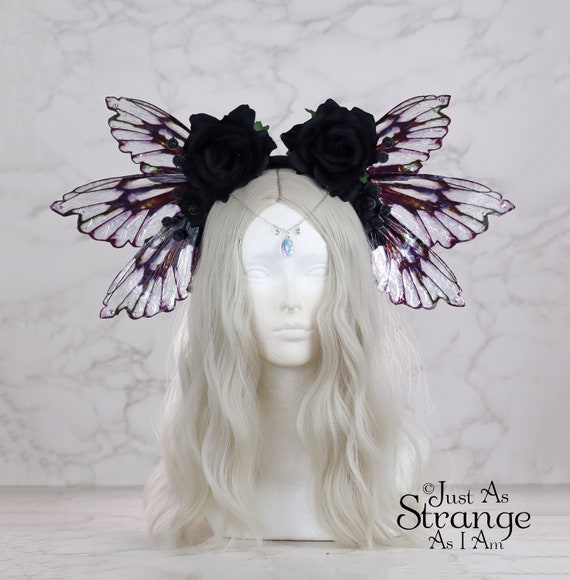The image showcases a pristine, eyeless, white mannequin bust positioned against a marble wall and resting on a marble surface, creating a monochromatic yet textured backdrop. The mannequin is adorned with a flowing, platinum blonde wig that cascades past its shoulders. Crowning the wig is an elaborate headpiece resembling butterfly wings, stretching widely from both sides and adorned with black roses. The headpiece features a mirrored headband with chains that dangle three drop crystals: a large, teardrop-shaped gemstone centered on the mannequin's forehead, flanked by two smaller round crystals on either side. These elements, together with the fantasy-like aesthetic, evoke a fairy costume. In the bottom right corner, the caption "Just as strange as I am" is elegantly inscribed in calligraphy, completing the whimsical and otherworldly theme of the advertisement.